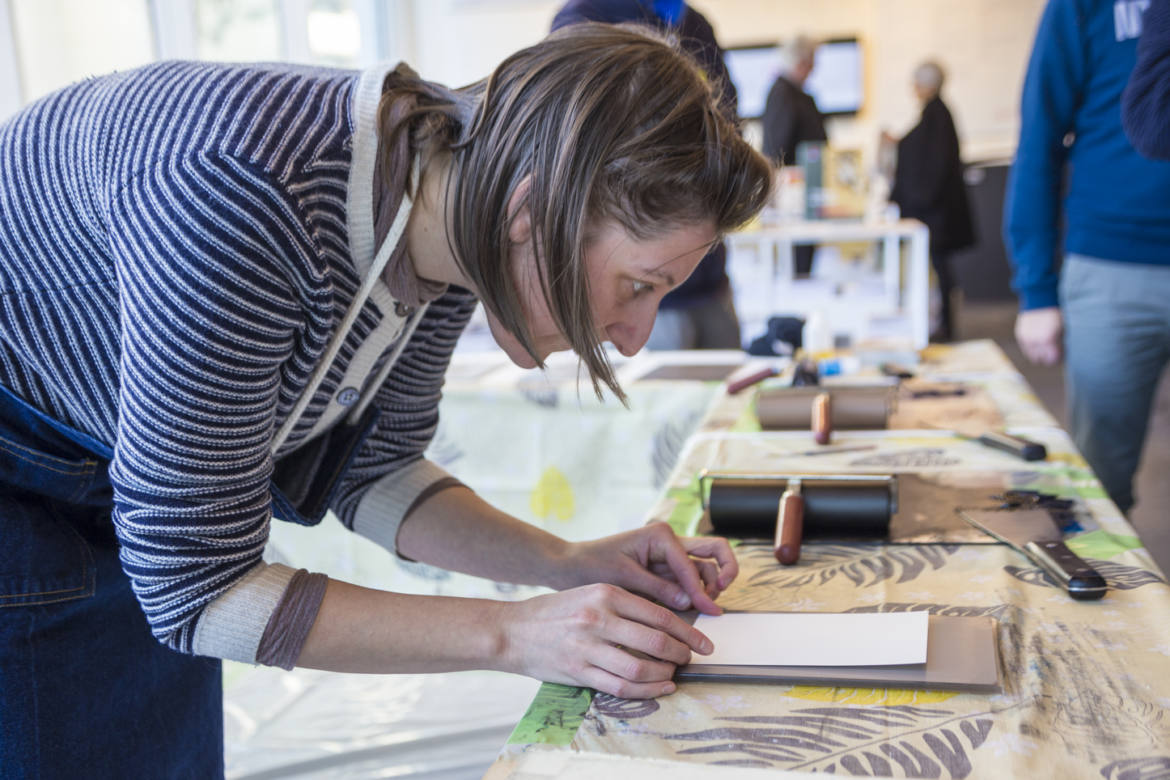In this photograph, a young woman in her 20s is deeply engrossed in a craft project at an event where crafts are either displayed or sold. She sits at an artistic table, working meticulously on what appears to be fabric printing. Her attire includes a blue and white striped sweater with blue buttons and a denim skirt; underneath, she wears a brown shirt. Her dirty blonde hair, somewhat stringy and pulled back with a barrette, falls around her face, indicating her complete focus on her work rather than her appearance. She is bent over, centering a white piece of paper on a brown canvas, surrounded by her tools: paint rollers, an ink roller, and a spatula. Blurred people in the background, wearing blue tops and black jackets, suggest that this scene takes place in a bustling public space, but they remain out of focus, emphasizing the woman's dedication to her craft.